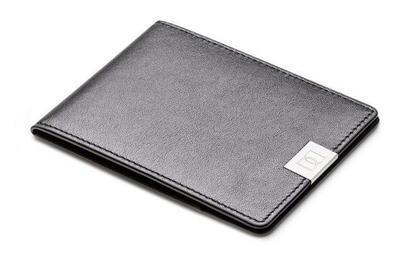The image depicts a slim black leather wallet positioned against a crisp white background. Captured from a slightly angled overhead perspective, the wallet showcases meticulously embossed black stitching along its edges. A notable feature is the silver metal enclosure on one side of the wallet's opening. This enclosure is a rectangular piece adorned with an engraved insignia formed by two overlapping capital letter D's, facing each other in a Venn diagram-like fashion. The clarity and brightness of the image highlight the wallet's luxurious detailing and craftsmanship.